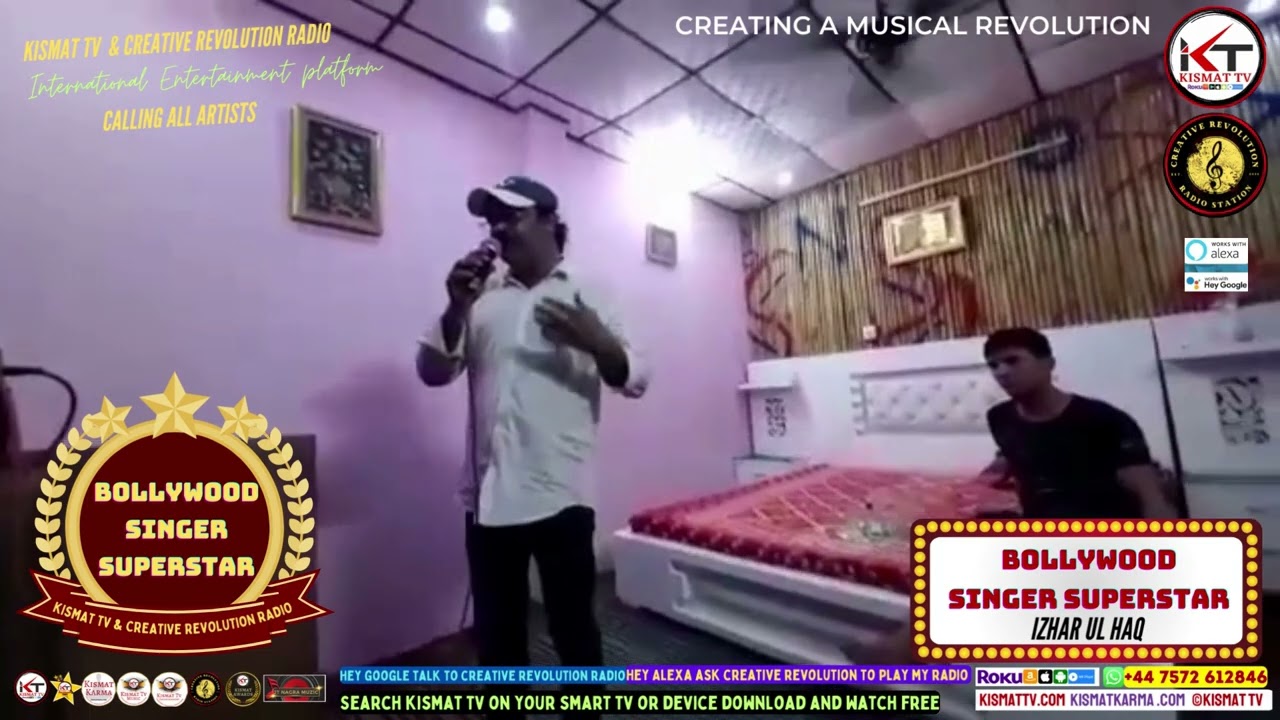This detailed image captures a scene from an advertising photograph for a TV program available on YouTube or similar platforms. The program is titled "Creating a Musical Revolution," broadcasted on Kismet TV and Creative Revolution Radio, and it specifically calls out to artists. In the foreground, an Indian man, adorned in a white shirt, black trousers, glasses, and a blue and white baseball cap, holds a microphone as if he is singing. A black-moustached man in a black t-shirt sits on a double bed with a red bedspread behind him, suggesting a casual, intimate setting, possibly a bedroom with purple walls and lacquered wood accents.

The room's ceiling appears to be made of rectangular padded tiles, and the floor is black. The bed has a unique red blanket featuring a diagonal geometric pattern, contributing to the vibrant yet homey atmosphere. Numerous text elements and logos frame the image. On the top left, it reads “Creating a Musical Revolution” and “Kismet TV and Creative Revolution Radio calling all artists.” The top right corner too states “Creating a Musical Revolution.” The bottom corners prominently feature the label “Bollywood Singer Superstar,” with the bottom left demonstrating a gold-bordered circular logo with stars and the bottom right showing a movie-themed symbol. 

Further down, the image displays various engaging options for viewers: “Hey Google, talk to Creative Revolution Radio,” “Hey Alexa, ask Creative Revolution to play my radio,” and “Search Kismet TV on your smart TV or device, download and watch for free.” Contact details including a phone number +447572612846, and several URLs such as KismetTV.com and KismetKarma.com are listed alongside the instructions. All these elements suggest this is an elaborate TV commercial aimed at launching or promoting a singing competition or talent show titled “Bollywood Singer Superstar,” aiming to create a substantial digital presence.